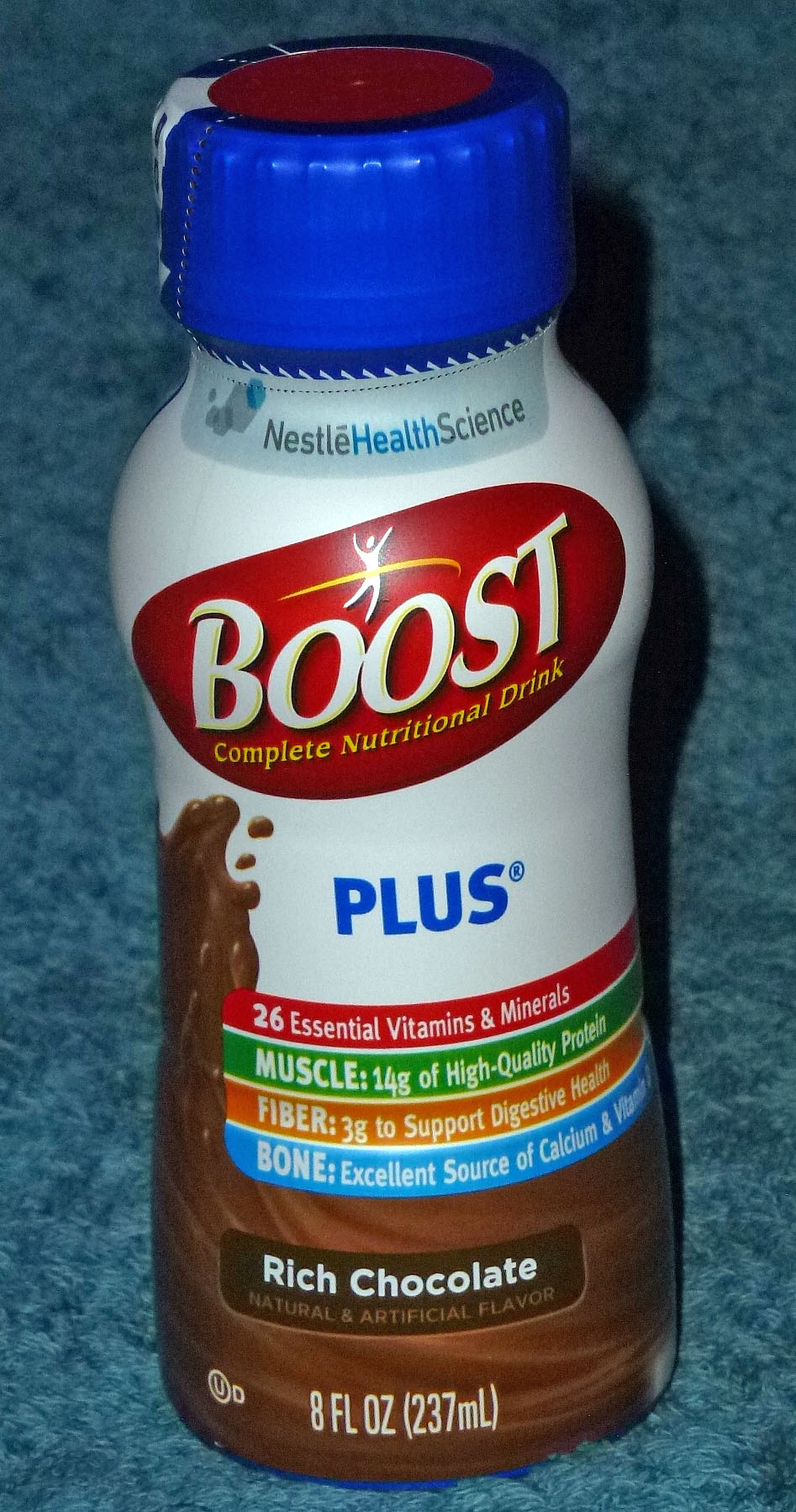This photograph showcases a bottle of Boost drink prominently placed on a blue carpet. The image is illuminated primarily by the camera's flash, casting a direct light on the subject. The bottle is sealed with a cobalt blue plastic cap. Central to the bottle's design is the label, which prominently features the "Nestle Health Science" logo at the top. Below this, the "Boost" logo is displayed in bold white font within a red oval shape.

Further down the label, the product is described in a yellow font as a "Complete Nutritional Drink." Directly beneath this description, the word "Plus" is highlighted in the same cobalt blue as the cap. The label further details the drink's benefits, stating it contains "26 essential vitamins and minerals," offers "14 grams of high-quality protein" for muscle support, provides "3 grams of fiber to support digestive health," and is an "excellent source of calcium and vitamin D" for bone health. The flavor of the drink is specified as "Rich Chocolate."

The detailed product information on the label emphasizes its nutritional benefits and positions the Boost drink as a comprehensive dietary supplement.